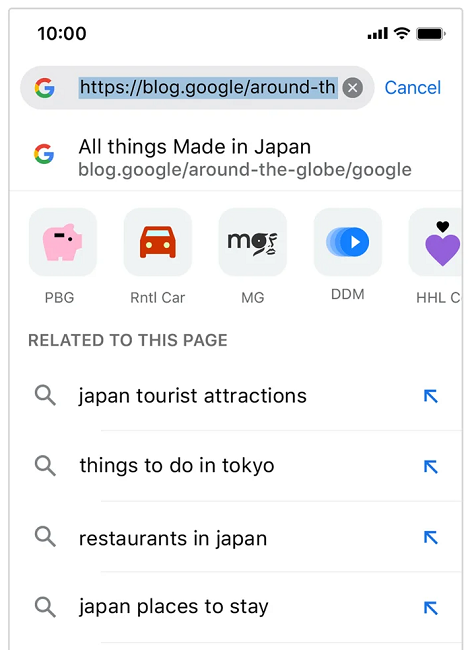This screenshot features a tablet displaying various on-screen elements. At the top left, bold black letters indicate the current time as 10:00. On the top right, icons display the signal strength, Wi-Fi status, and battery level.

Below the status bar is a search bar with the Google "G" logo on the left. Within the search bar, the partially typed URL "HTTPS://BLOG.GOOGLE//AROUND//TH" appears, and on the right side of the search bar is a blue "Cancel" button.

Underneath the search bar is another Google "G" logo followed by the search result title "All things made in Japan" and the URL "HTTPS://BLOG.GOOGLE//AROUND//TH//GLOBE//GOOGLE".

The next section displays five square icons, each with accompanying text below them. The first icon depicts a pig and is labeled "PBJ". The second box shows an icon labeled "CARB" with the text "RNTL CARB" underneath. The third icon, featuring a stylized "M" and squiggly lines, is titled "MG". The fourth box contains a circle with a triangle pointing to the right, titled "DDM". The final box showcases a purple heart overlaid with a smaller black heart and is labeled "HHLC".

Beneath these icons is a section titled "Related to this page," listing four search items: "Japan tourist attractions," "Things to do in Tokyo," "Restaurants in Japan," and "Japan places to stay".